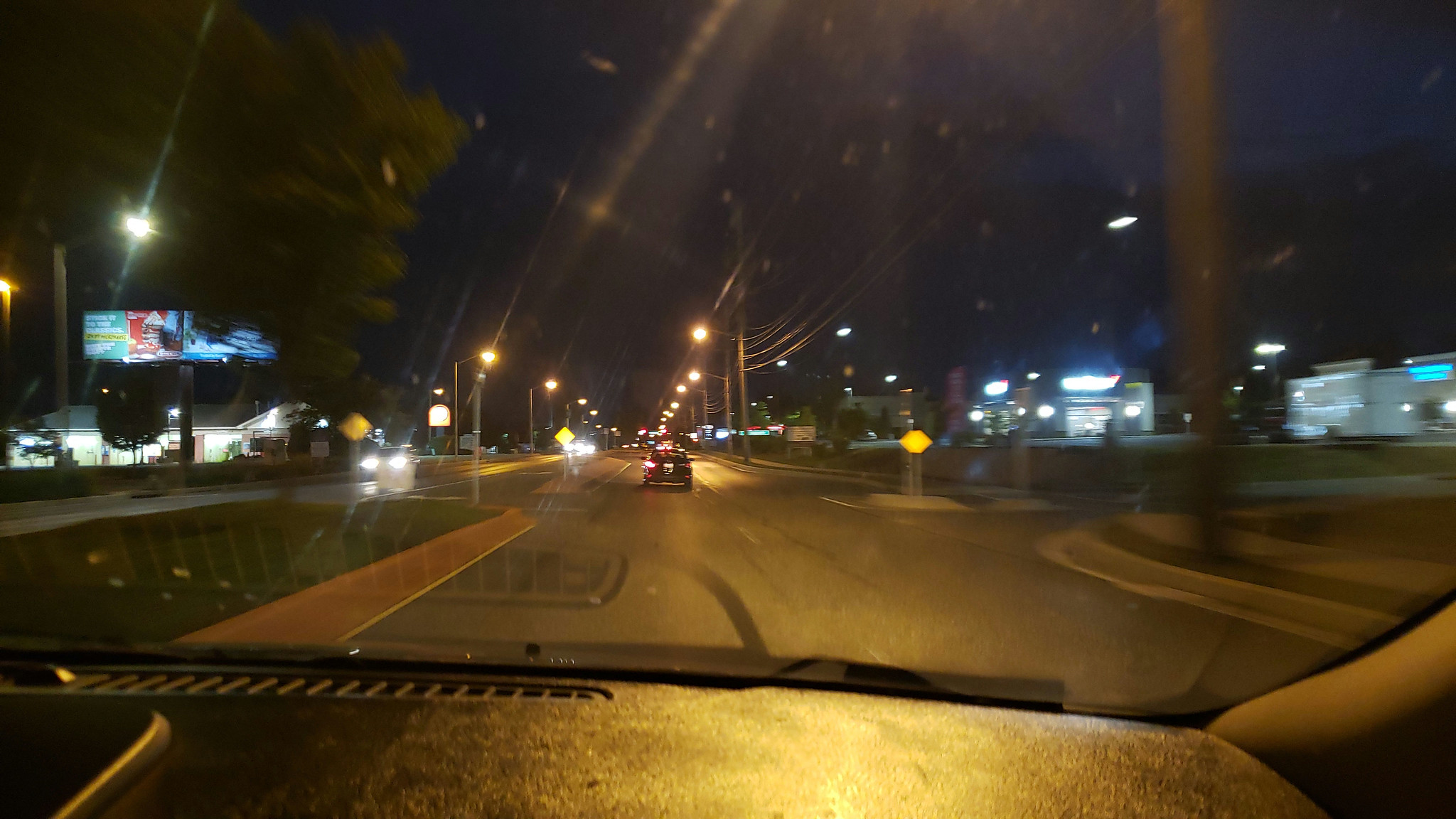The image depicts a nighttime scene captured from the inside of a car, taken through the front windshield, which shows dirt specks and reflections. The dashboard is visible along the bottom of the photograph. The vehicle is traveling in the left lane of a divided highway, with a grassy median to the left bordered by a wide curb, and another empty lane to the right. The road surface appears damp, possibly due to recent rain.

In the distance, a dark-colored sedan is visible, potentially with one taillight out, shining a light pinkish hue from its left taillight. There is oncoming traffic in the opposite lanes, with headlights piercing the dark night. Streetlights and utility poles line both sides of the road, with a receding line of glowing orbs from the illuminated street lamps guiding the way. Larger trees loom overhead on the left side of the road, including a substantial green oak tree, while the right side features smaller trees and a series of national and local businesses.

Billboards are scattered along the roadway, one notably showing a red background with food, while others are too blurry to discern clearly. Yellow caution or speed limit signs, glowing from reflected light, are positioned along the median, the right side of the road, and the opposite lane.

The right side of the road features various buildings, including a condo-like structure, corporate buildings with lit signage, and a series of storefronts resembling a strip mall development. One of the buildings has an aqua blue illuminated sign, while another's signage remains indistinct due to blurriness. Beneath this assortment of structures, sidewalks and curbing with grassy patches add to the suburban feel of the setting.